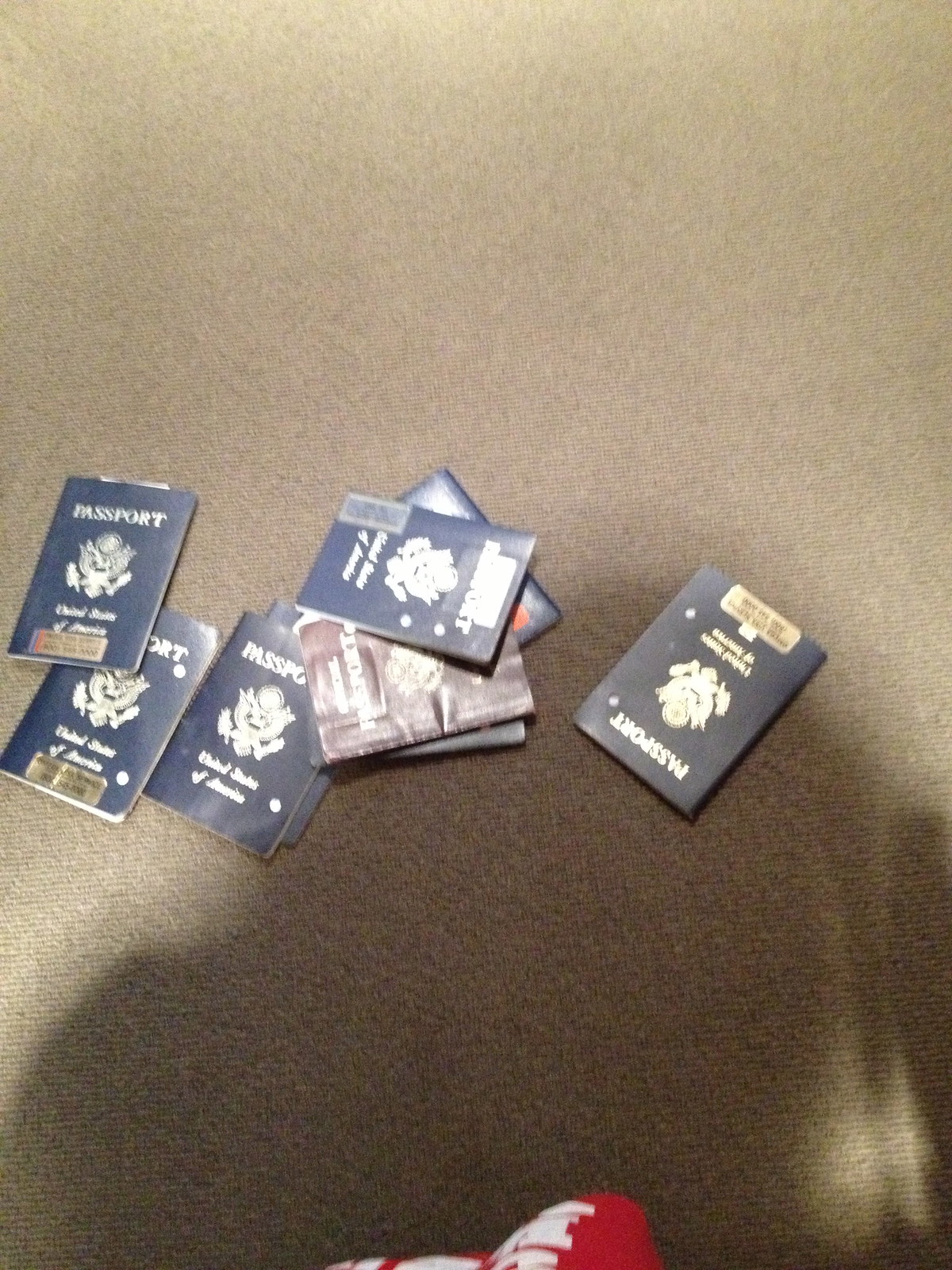This image captures a scattered arrangement of nine passports sprawled across a poorly maintained brown carpet. Most of the passports—eight to be precise—are uniform in appearance with dark blue covers. Each of these blue passports prominently displays "PASSPORT" in white above an emblem of an eagle clutching an olive branch and arrows, along with "United States of America" inscribed below. In stark contrast, at the center of the group, a lone passport with a worn and wrinkled cover in a faded reddish-brown hue stands out amidst the others. The composition shows four passports stacked centrally, with four more to the left and a single passport positioned at the bottom right. The bottom section of the photograph is partially overshadowed, possibly by the photographer, with a hint of red, attributed to an object or element not part of the passport collection.